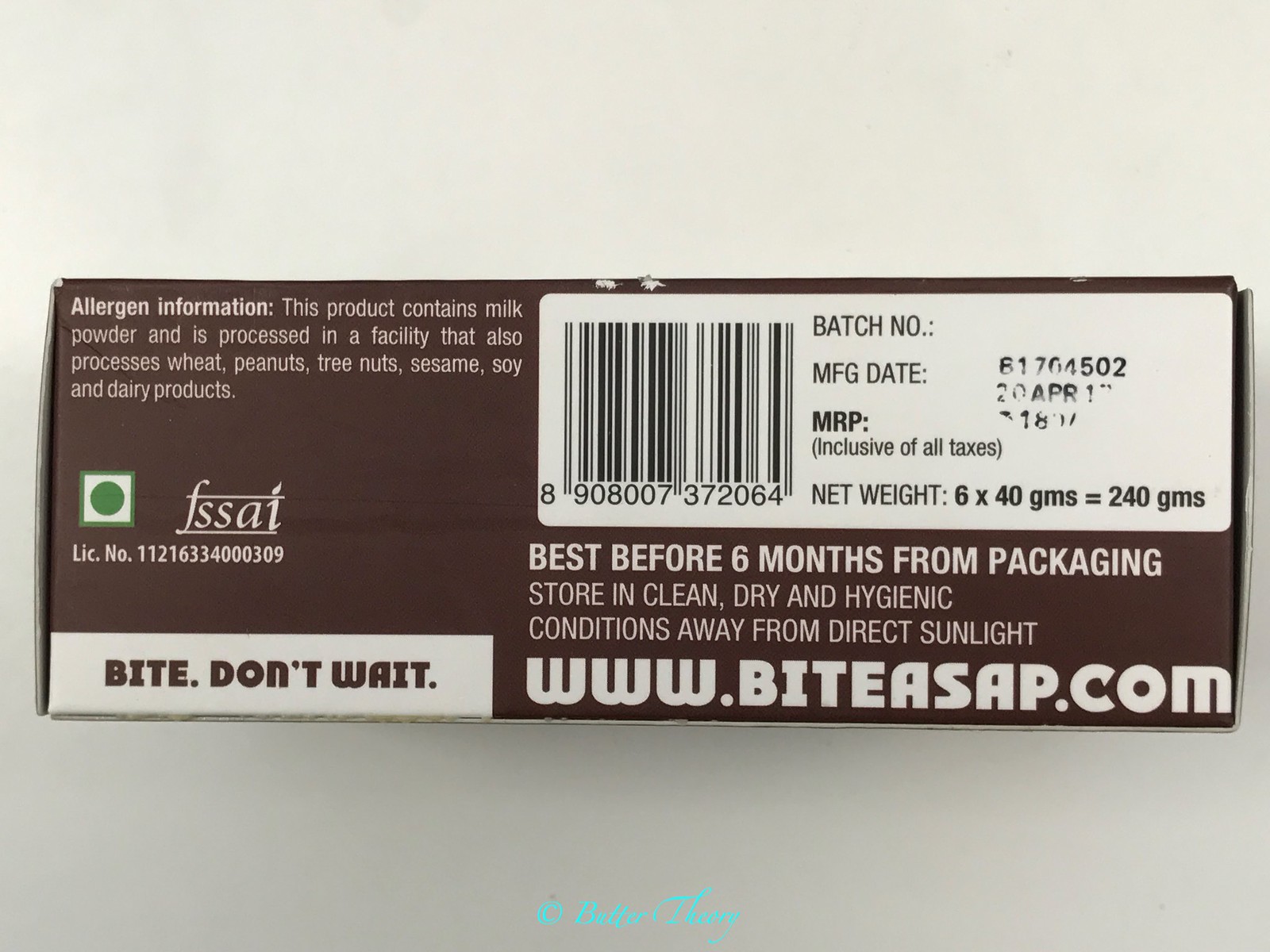The image displays a pale grey rectangular package featuring a centrally located, dark brown or black label. The label includes white lettering and a prominent white section that holds a barcode, manufacturing dates, and other relevant information, such as the item's weight. It also indicates that the product is "Best before six months from packaging." 

Beneath this information, the label advises to "Store in clean, dry, and hygienic conditions away from direct sunlight." Additionally, a website link, "www.biteasap.com," is provided on the right side of the label. On the left side, there is a white lozenge-shaped section with the text "Bite. Don't wait" inscribed inside. 

Above this lozenge, a green square encloses a white square, which itself contains a solid green circle. Inside this green circle are the letters "FSSAI" with an accent over the 'I', and a license number. Further up, allergen information is provided: "This product contains milk powder and is processed in a facility that also processes wheat, peanut, tree nuts, sesame, soy, and dairy products."

Overall, the meticulous packaging details suggest that this is a food product, but the long shelf life of up to six months after packaging may raise concerns about its freshness.